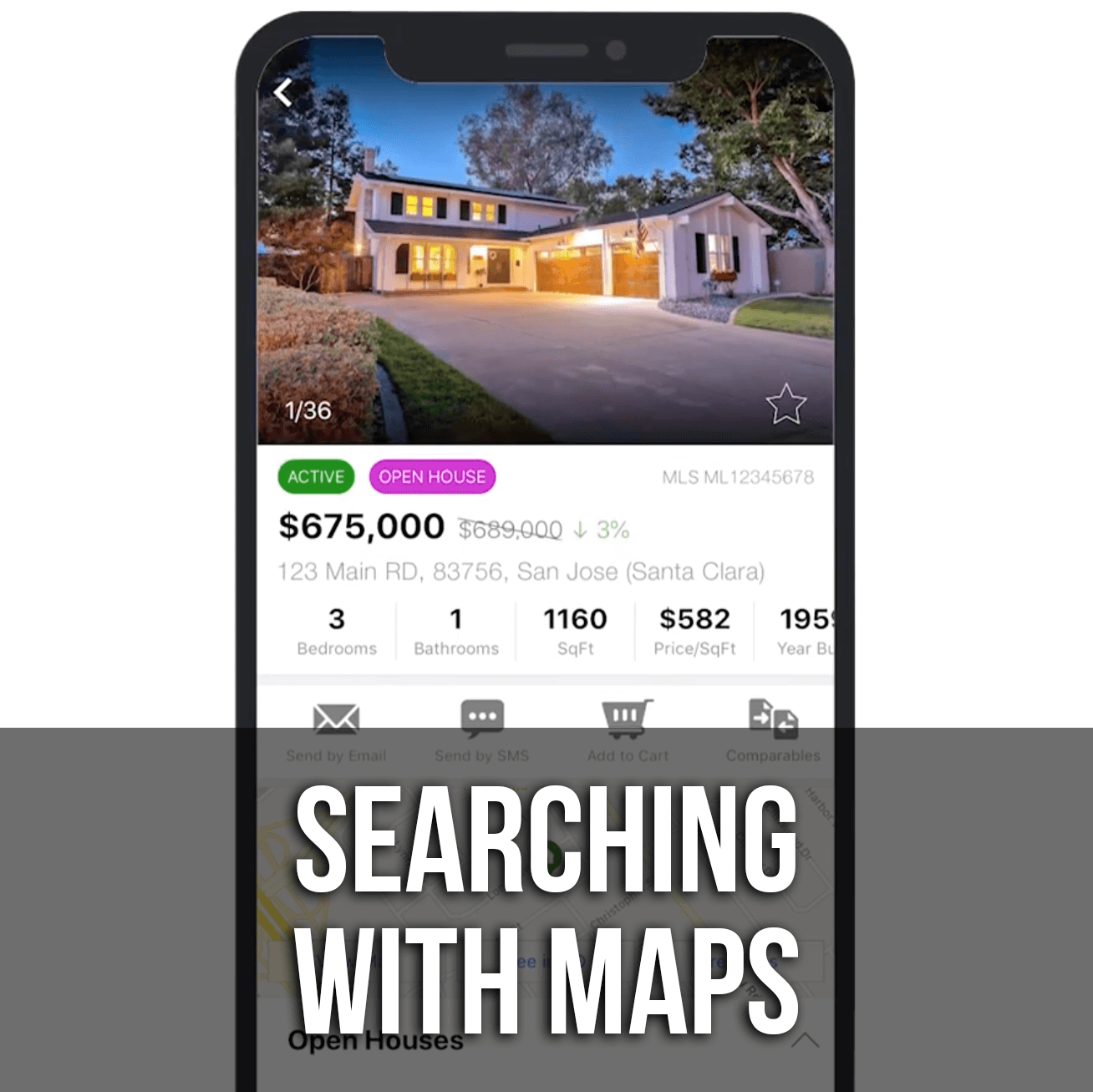Screenshot of a website or app functionality test displaying a mock phone interface. At the top of the screen, there is an image of a house taken around evening time. Below the image, the house's current price is shown as $675,000, and the previous price of $689,000 is crossed out with a diagonal grey line, indicating a price drop. Accompanying this, a downward arrow and a note of "3%" signify the percentage reduction in the price. The address of the property is detailed as "123 Main Road, San Jose, Santa Clara." Additional property details include: 3 bedrooms, 1 bathroom, totaling 1160 square feet of living space, and the price per square foot is listed as $582.